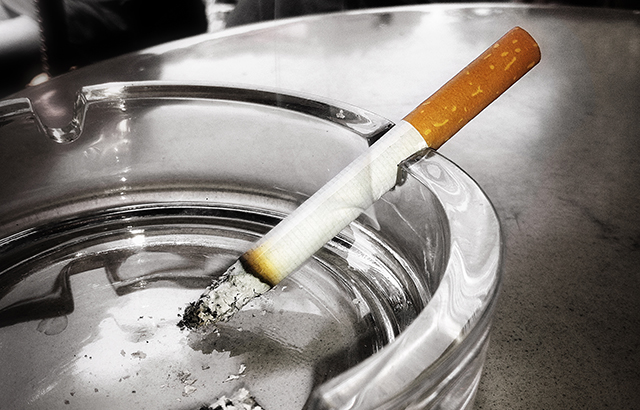This is an exceptionally high-quality close-up photograph of a traditional cigarette resting in a crystal-clear glass ashtray. The cigarette features a light brown filter with white specks, transitioning to a white main body that is half-burnt, revealing dark burn marks and white ash at the tip. The cigarette is nestled in one of the notched grooves of the ashtray, positioned on the right side. The ashtray itself, placed on the left side of the image, is meticulously clean, containing only a small amount of loose ash, suggesting minimal use. The setting is on a shiny, grayish-silver table, which emphasizes the clarity and pristine condition of both the cigarette and the ashtray. The photograph's close-up nature does not provide context for the surrounding environment, leaving the specific location ambiguous.